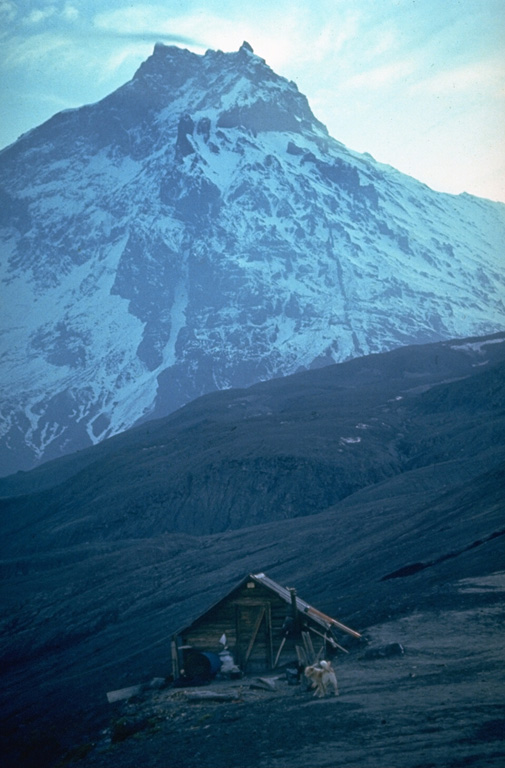The photograph captures an outdoor scene dominated by two mountains under natural, albeit poor, daylight. The vertically rectangular image features a towering, snow-covered, rocky mountain that occupies the upper half, with patches of dark gray rock interspersed among the white snow. The very top edge of the photo shows a sliver of blue sky with faint white clouds. 

In contrast, the bottom half of the image presents a smaller, darker mountain, composed of brown and dark gray rocky terrain. Nestled at the base of this mountain is a tiny, weathered wooden shack with a triangular, A-frame style roof, which appears to be made of metal. The door is nearly as tall as the roof’s peak, constructed from dark brown wood. Outside this modest structure, which is barely larger than a tent, wanders a yellow dog, adding a touch of life to the rugged landscape.